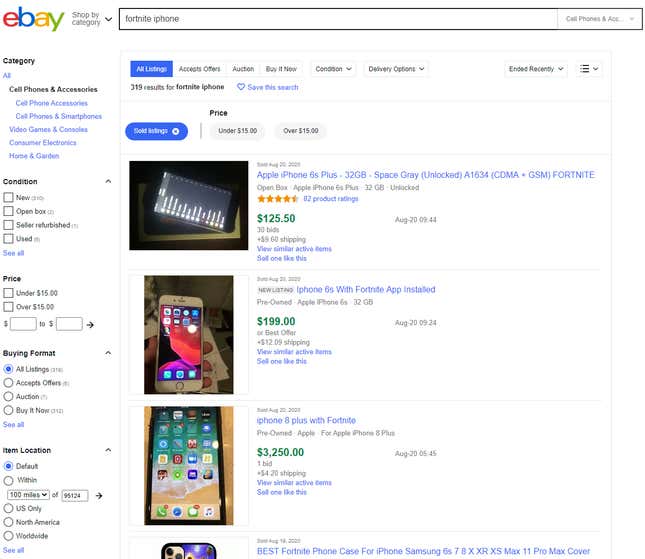**Detailed Caption for Screenshot of eBay Search Results Page**

This is a detailed screenshot of an eBay search results page, highlighting a search for "Fortnite iPhone." At the top left, the iconic eBay logo is visible in red, blue, yellow, and green. Below it is a "Shop by category" drop-down menu. 

The search query "Fortnite iPhone" is displayed prominently. To the right, a category filter is set to "Cell Phones & Accessories." There's an option to further refine this category through a drop-down menu.

On the left-hand side of the page, a comprehensive navigation menu typical of eBay is visible. It starts with broad categories like “Cell Phones & Accessories,” subdivided into more specific ones including "Cell Phone Accessories," "Cell Phones & Smartphones," "Video Games & Consoles," "Consumer Electronics," and "Home & Garden." Underneath these categories, there is a "Condition" filter with choices such as "New," "Open Box," "Seller Refurbished," and "Used," each with an option to "See All." Specific quantities for available conditions are listed here as well.

Price filtering options allow users to specify ranges or choose between "Under $15" and "Over $15." Additional options include the buying format, such as "All Listings," "Accepts Offers," "Auction," and "Buy It Now." Location settings default to within 100 miles of the 95124 zip code, but users can opt for broader regions like "U.S. Only," "North America," or "Worldwide."

To the right, within a gray-outlined box, "All Listings" are highlighted in blue. Filter options include "Accepts Offers," "Auction," "Buy It Now," "Condition," and "Delivery Options." A "319 results for Fortnite iPhone" tag is visible, with an option to save this search in blue text.

A menu to sort the listings by different criteria such as recently ended auctions is also displayed. Listings themselves feature various descriptions and prices. For instance, an iPhone 6S with the Fortnite app installed is listed as open box, priced at $125.50 with 30 bids, plus $15.60 shipping, ending August 20, 2009. Another listing contains a pre-owned Apple iPhone 6S 32GB for $199.00 or best offer, plus $12.09 shipping.

The listings continue with items like an iPhone 8 Plus featuring Fortnite, with a current bid at $3,250.00, $45.00 shipping, and one bid placed as of August 20, 2009. The very top listing highlights a "Best Fortnite phone case for iPhone 6S, 7, 8, X, XR, XS, Max, 11 Pro Max cover".

Each listing includes options in blue text to view similar active items or to sell one like it. Various thumbnails of the products are displayed, with the items often shown in a horizontal orientation. Overall, the filtered and structured results provide a user-friendly experience for buyers looking for Fortnite-related iPhone products on eBay.